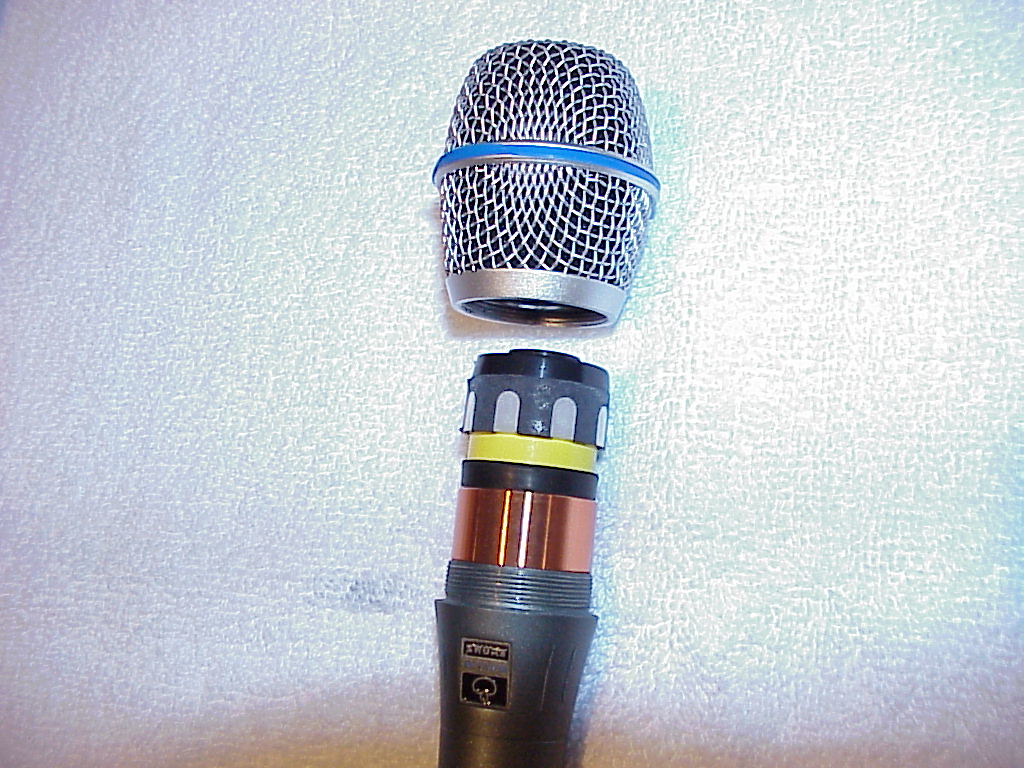The photograph features a disassembled microphone, positioned in the center of the image, resting on a textured and slightly fraying white terry cloth towel. The towel is brighter on the right side, with shadows filling the corners and a small hole forming to the left of the microphone. The microphone is in two pieces: the head and the base. The head, displaying internal components, is situated just above the handle in the middle of the image. The handle, partially visible at the bottom, flaunts a small, somewhat indistinct black logo with a silver border. The internal components of the microphone are sequentially highlighted by a copper band, followed by black, yellow, and gray bands. The microphone head itself is primarily silver with a distinctive blue band encircling its center. The overall color palette includes blue, gray, copper, yellow, black, and white, all harmonized against the backdrop of the white towel.